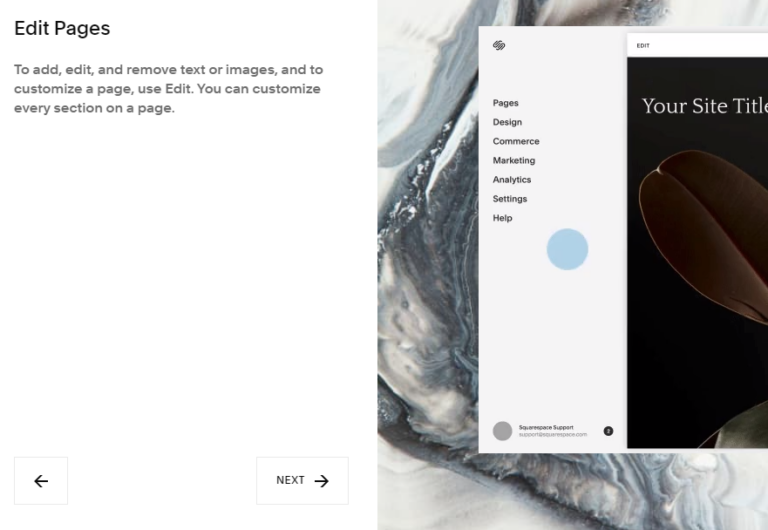The image displays a user interface for webpage customization, set against a white background. On the left side, there's a black sidebar with options to "Add," "Edit," and "Remove" text or images, allowing for extensive page customization. This sidebar also includes a black back arrow encased in a white box, as well as another white box containing a black "Next" icon with an arrow. To the right in the main section of the interface, there's a close-up view of a silver and white object, partially covered by a white box showing a brown object with black text.

At the top of the interface, there's a black icon resembling a fingerprint, alongside menu options like "Pages," "Design," "Commerce," "Marketing," "Analytics," "Settings," and "Help." A blue circle is also subtly visible in this area. Towards the bottom, there is some gray text accompanied by a gray circle, and a dark-colored box featuring white text. Overall, the image quality is decent, but the smaller gray font near the circle is hard to read due to its size.